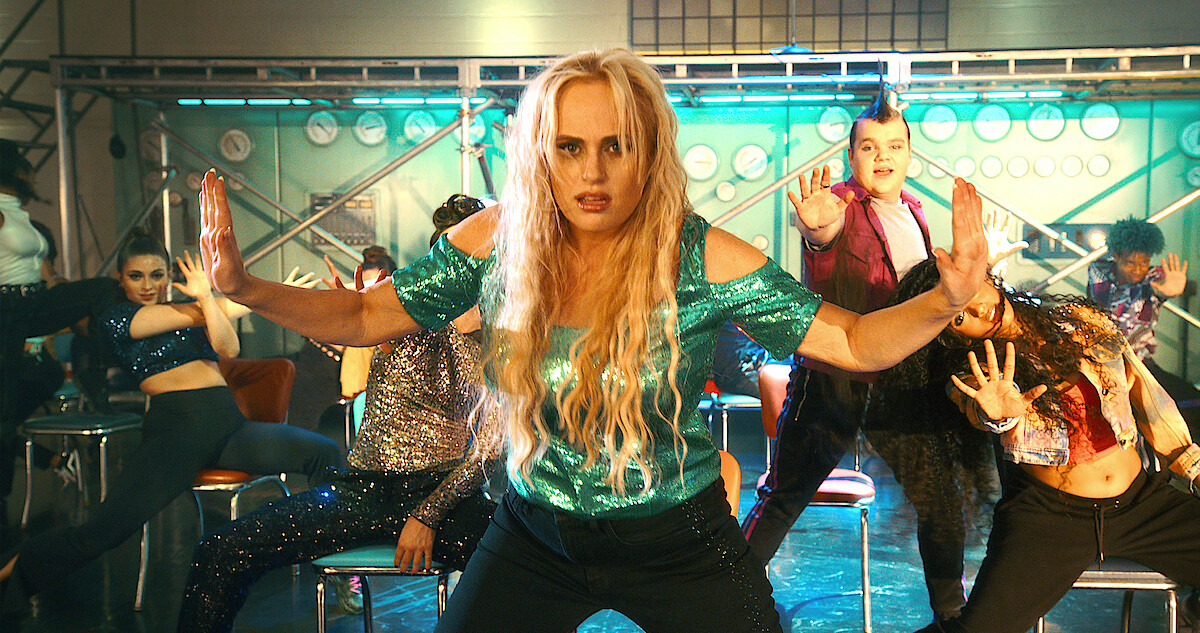In this vibrant scene from a movie, Rebel Wilson, the focal point, stands confidently with her arms outstretched in an expressive stance. Clad in a sparkly green top and black pants, her long blonde hair frames her face radiantly. She is surrounded by a lively ensemble of men and women, engaged in a dance routine. The background is a dynamic stage setup, adorned with theatrical lights, scaffolding, and clocks. Some performers are striking poses while balanced on thin metal-rail chairs reminiscent of the 70s, their flashy red and other colorful outfits adding to the energetic ambiance. The blue floor accentuates the visual appeal, capturing a lively and dramatic moment from the performance.